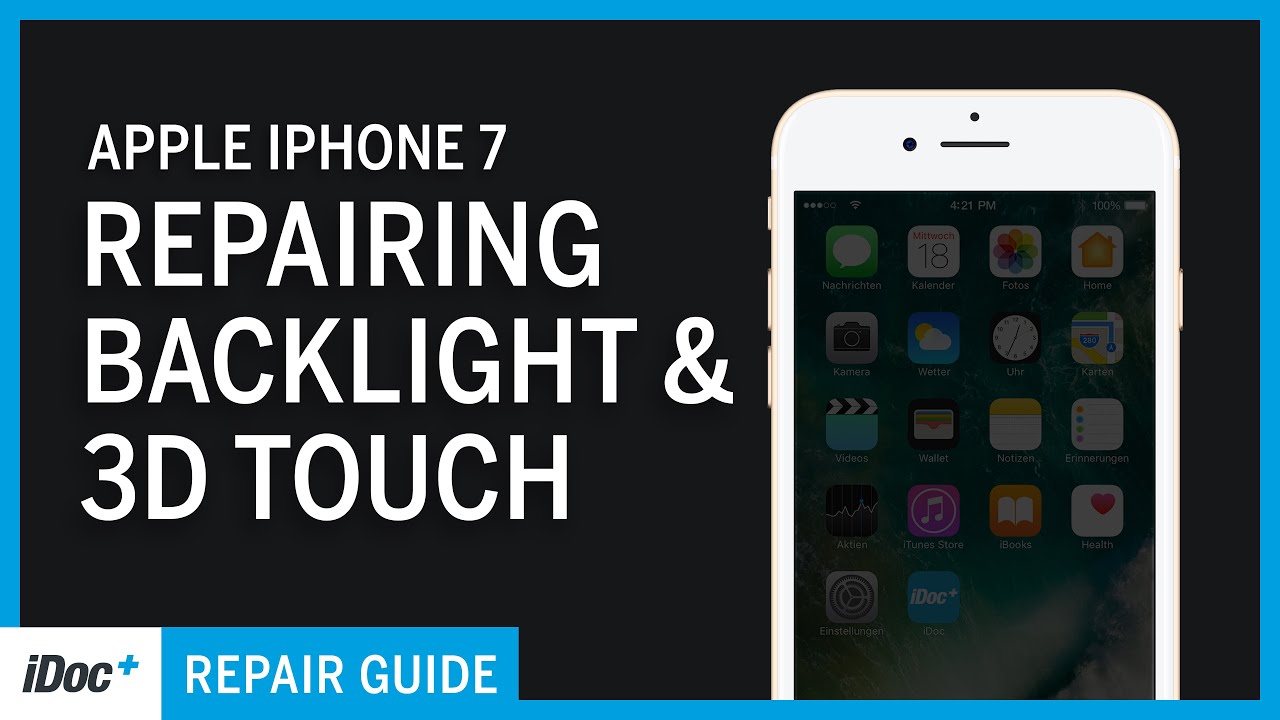The image is a rectangular graphic advertisement with a light blue skinny border and a black background. Prominently displayed in bold white font are the words "Apple iPhone 7 Repairing Backlight and 3D Touch." In the bottom left corner, the text reads "iDoc Plus Repair Guide," accompanied by a small blue square with the words "Repair Guide" in white. The right side features a top-half view of a white iPhone 7, recognizable by its relatively big bezels and absence of a notch. The phone's screen displays a faded, not well-lit traditional home screen with various app icons. This advertisement suggests a self-repair guide for common issues, specifically focusing on the backlight and 3D Touch, aimed at helping users perform repairs themselves instead of opting for potentially expensive professional services.